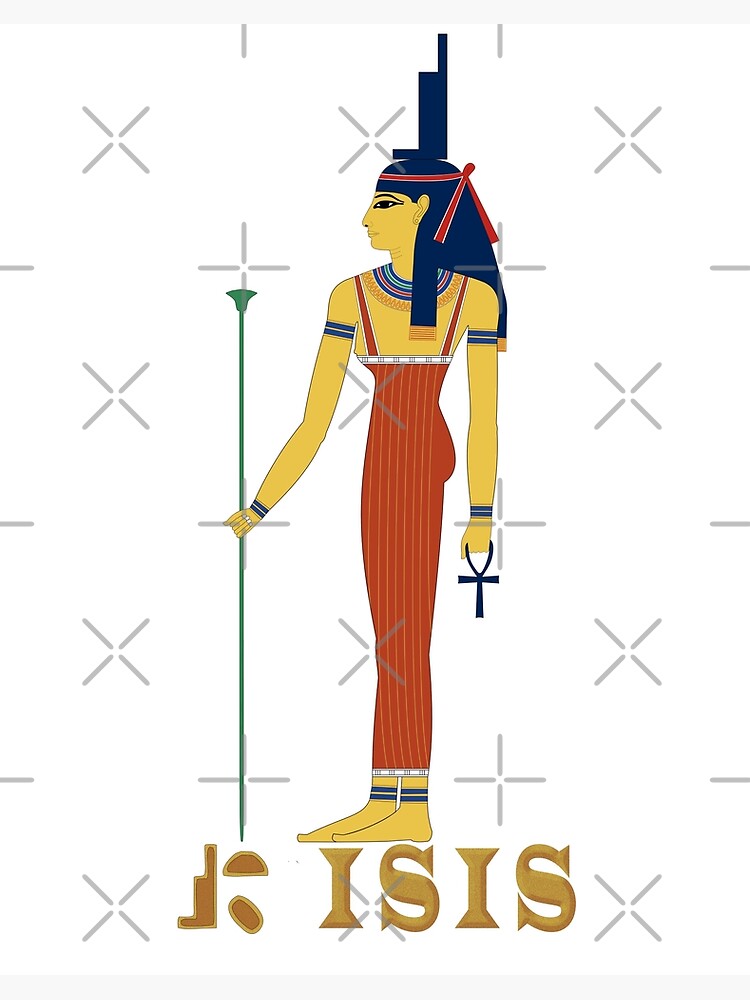The image features a detailed artistic representation of the Egyptian goddess Isis, set against a white background adorned with a complex watermark consisting of grey X's, plus signs, and dashes, creating a layered pattern with a white spot at the center. Isis is depicted with geometric, navy blue hair, perfectly flat at the bottom and adorned with a red band. She has large, horizontally elongated eyes and wears a striking red dress complemented by necklaces around her neck. Her skin is depicted in gold, covering her arms, legs, and feet. In her left hand, she holds an ankh, the Egyptian symbol for life, while her right hand grasps a long, green scepter that extends to the ground. At the bottom of the image, the name "ISIS" is written in dark gold letters, along with hieroglyphs indicating her divine identity. Isis stands facing the left, completing this classic piece of Egyptian-themed artwork.